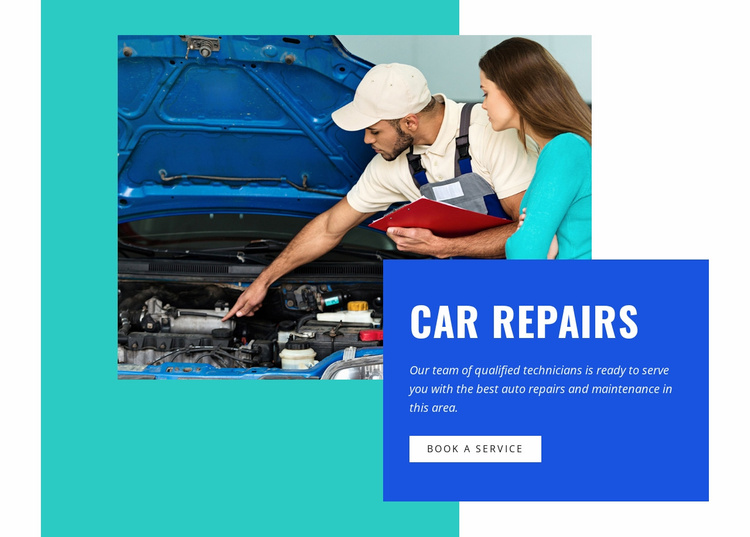The image is a screenshot from a website, featuring a predominantly turquoise background on the left and middle sections. Towards the center, slightly offset to the left, there is a photograph or graphic displaying a car with its hood up, revealing the engine compartment. A man dressed in a white t-shirt, overalls, and a white cap styled like the Facebook logo is pointing to a specific part under the hood. He is holding a folder in his left arm. 

Standing next to him, to his left, is a woman with dark, long hair. She is partially visible from her left side, with her arms crossed, attentively looking at the area the man is indicating under the hood.

Beneath the woman's torso, there is a blue square with large white text that reads "Car Repairs." Below this, a smaller white rectangle contains the text: "Our team of qualified technicians is ready to serve you with the best auto repairs and maintenance in this area." Further down, another white rectangle has a call-to-action message, "Book a Service."